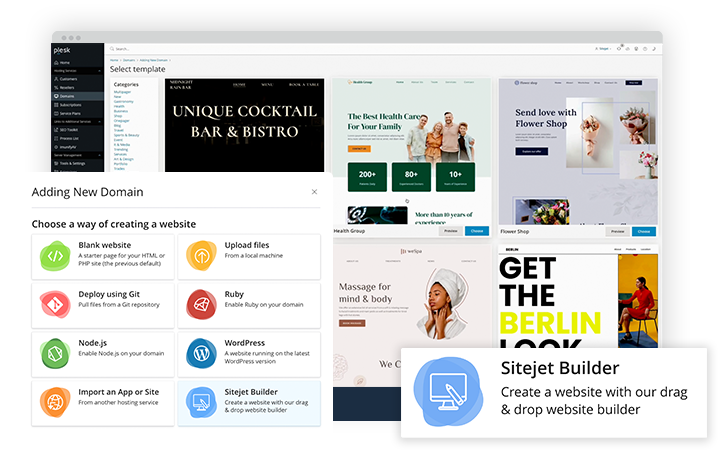The image depicts a user interface screen for a web page creation platform named SiteJet Builder. The screen is filled with various advertisements and options dedicated to website design and deployment. On the right side of the interface, the brand "SiteJet Builder" is prominently displayed at the bottom, accompanied by a blue shape that features a white outline of a computer monitor and a pencil, symbolizing website creation tools.

The interface offers a selection of templates and methods to create a website. Users can choose different methods shown via colored buttons, each representing distinct features such as creating a blank website, uploading files, and deploying using GIT. Other options include frameworks and platforms like Ruby, Node.js, WordPress, and importing an Apple site. Notably, WordPress is mentioned as a familiar word processing system. Additionally, there are various example websites displayed toward the right-hand side and at the top of the screen, demonstrating possible outcomes and templates available for users to select from.

Overall, the image clearly represents a robust web page creation tool aimed at making website design accessible, customizable, and efficient for users.